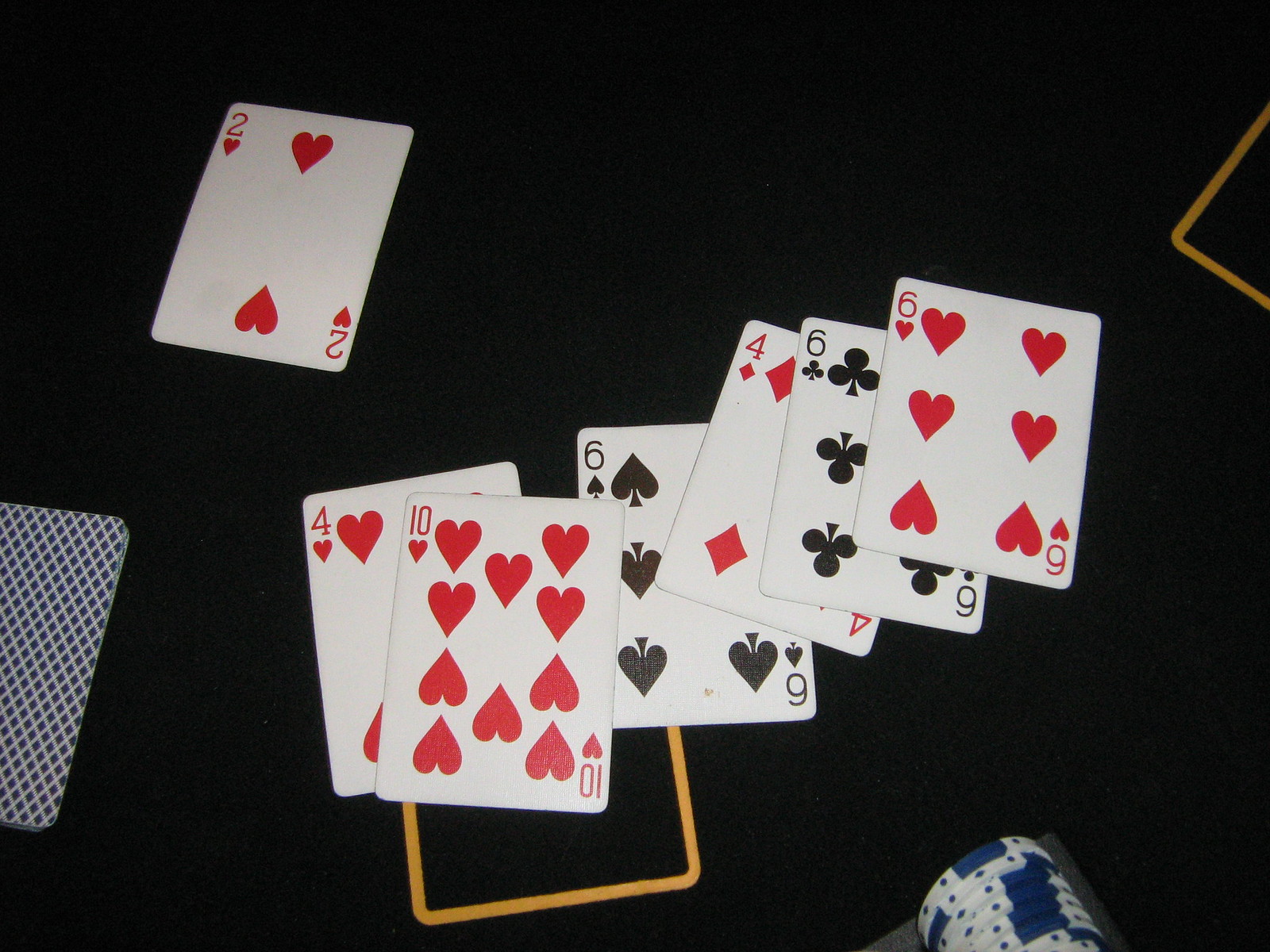An overhead view photo captures a dynamic poker scene on a black poker table adorned with gold-bordered rectangles for card placement. At the center, six playing cards are prominently displayed, all face up. Positioned at the top left, a Two of Hearts takes an angled stance. Below, from left to right, a Four of Hearts partially overlaps with a Ten of Hearts. Adjacent to these, a Six of Hearts, a Four of Diamonds, and a Six of Clubs are all angled towards the right. Notably, another Six of Hearts is also angled in the same direction. The background of the table features a striking blue with white X’s pattern, seen on the backs of additional cards partially visible in the bottom left corner, face down. In the bottom right, stacks of blue and white poker chips are neatly organized in a tray, adding to the competitive ambiance of the game.